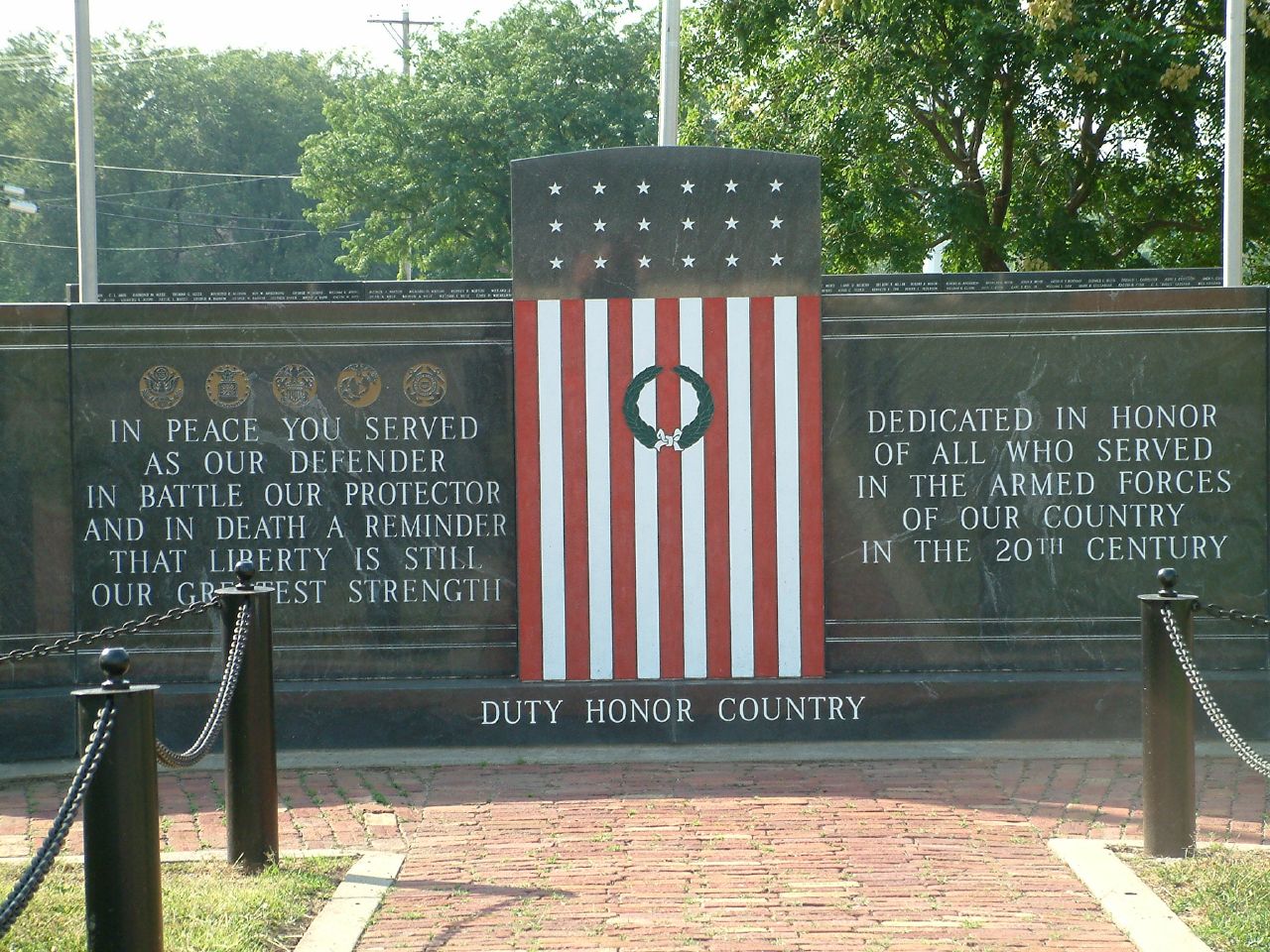The photograph captures an outdoor memorial set against a backdrop of trees and vegetation, bathed in natural daylight. At its center is a polished black stone wall featuring an American flag rendered in stone. The flag hangs vertically, with its top portion crafted from a plain metal bearing 18 stars, and the bottom composed of vertically colored red and white stripes, accentuated by a green wreath in the center. Inscribed on the left side of the wall are the words: "In peace you served as our defender, in battle our protector, and in death a reminder that liberty is still our greatest strength." To the right, another inscription reads: "Dedicated in honor of all who served in the armed forces of our country in the 20th century." Below the flag, the phrase "duty, honor, country" is prominently displayed. A red brick pathway leads up to the memorial, bordered by a manicured lawn and a black chain-link fence supported by posts. Shadows from the posts and the vegetative surroundings suggest the photo was taken during the daytime.